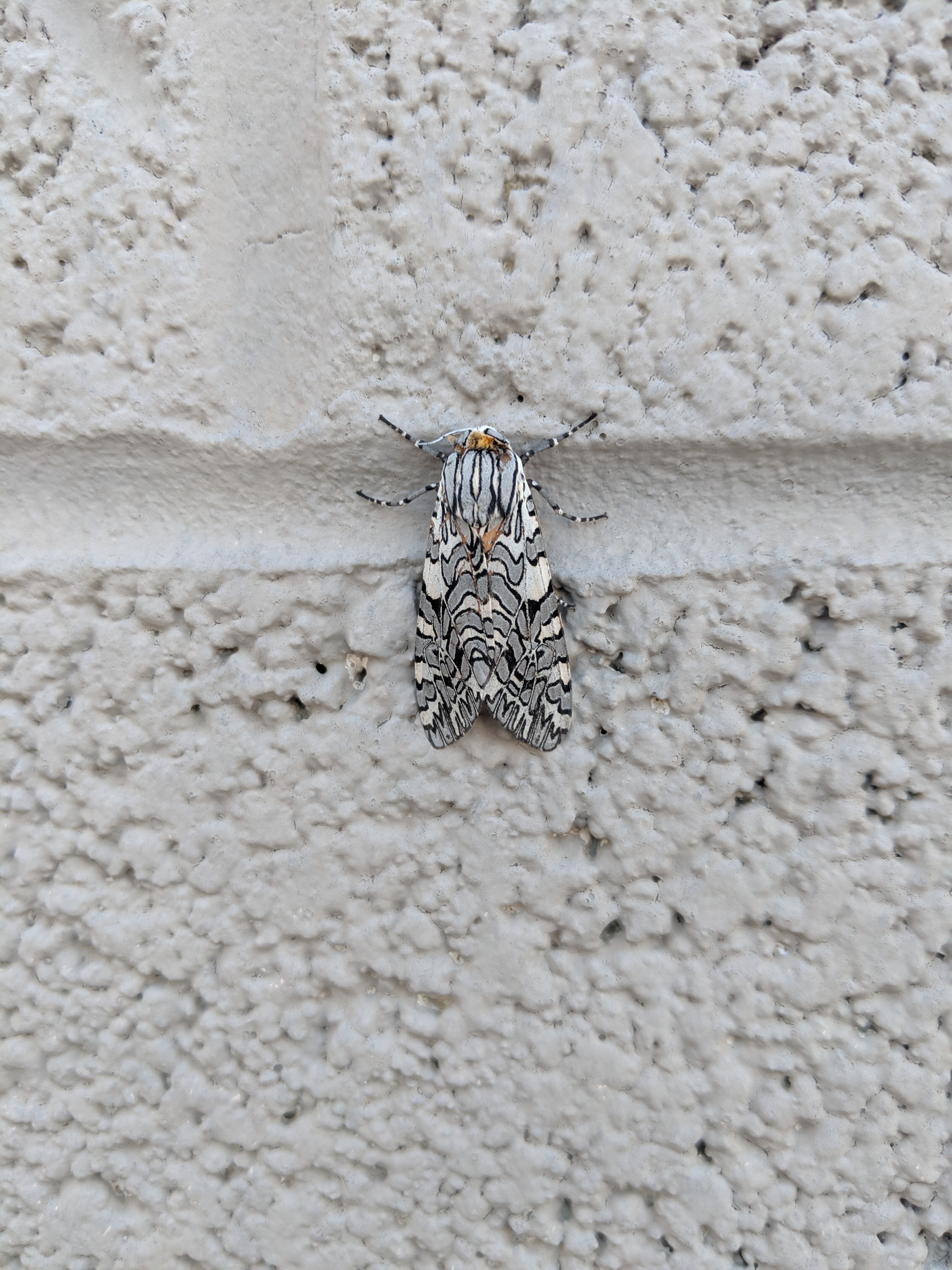This incredibly detailed macro photograph captures a striking insect resting on the white-painted surface of a textured concrete wall. Positioned on the grout line between two blocks, the insect is adorned with an intricate pattern of black, white, and gray stripes, creating a mesmerizing display across its wings, body, and slender legs. The bug, potentially a moth, features a complex wing design that combines diamond and oval shapes outlined in black. While its wings are folded back, they dominate its small, approximately one-inch frame. Additionally, the insect showcases subtle touches of muted orange on its head and back, and its delicate white antennae add to its intricate appearance. The concrete wall's thick, white paint offers a stark contrast to the bug's detailed patterns, making it a standout subject in this realistic and vivid close-up image.